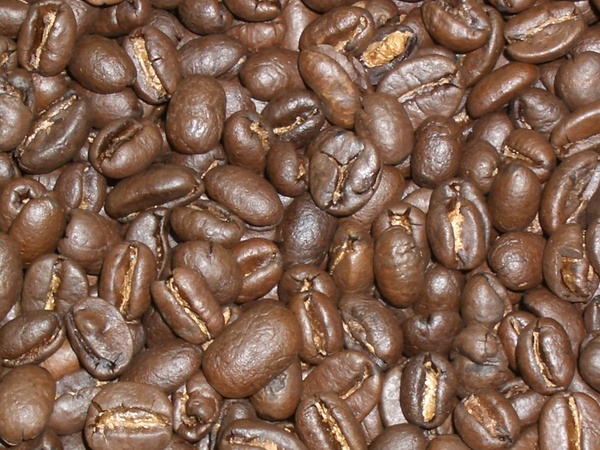This close-up photograph showcases a large pile of dark, chocolatey-brown roasted coffee beans, filling the entire frame of the rectangular image, which measures approximately 4 to 5 inches wide and 3 inches high. The coffee beans are small, elliptical, and vary in orientation—some upright, some upside down, and others sideways. Each bean features a distinguishing light brown slit running lengthwise, revealing a light tan-colored interior. The beans are depicted in various stages of splitting open. The image is brightly lit, with no noticeable dark shadows, giving a clear and detailed view of the textured surfaces of the coffee beans, all laying contiguously, suggesting they might be inside a bag or sack.